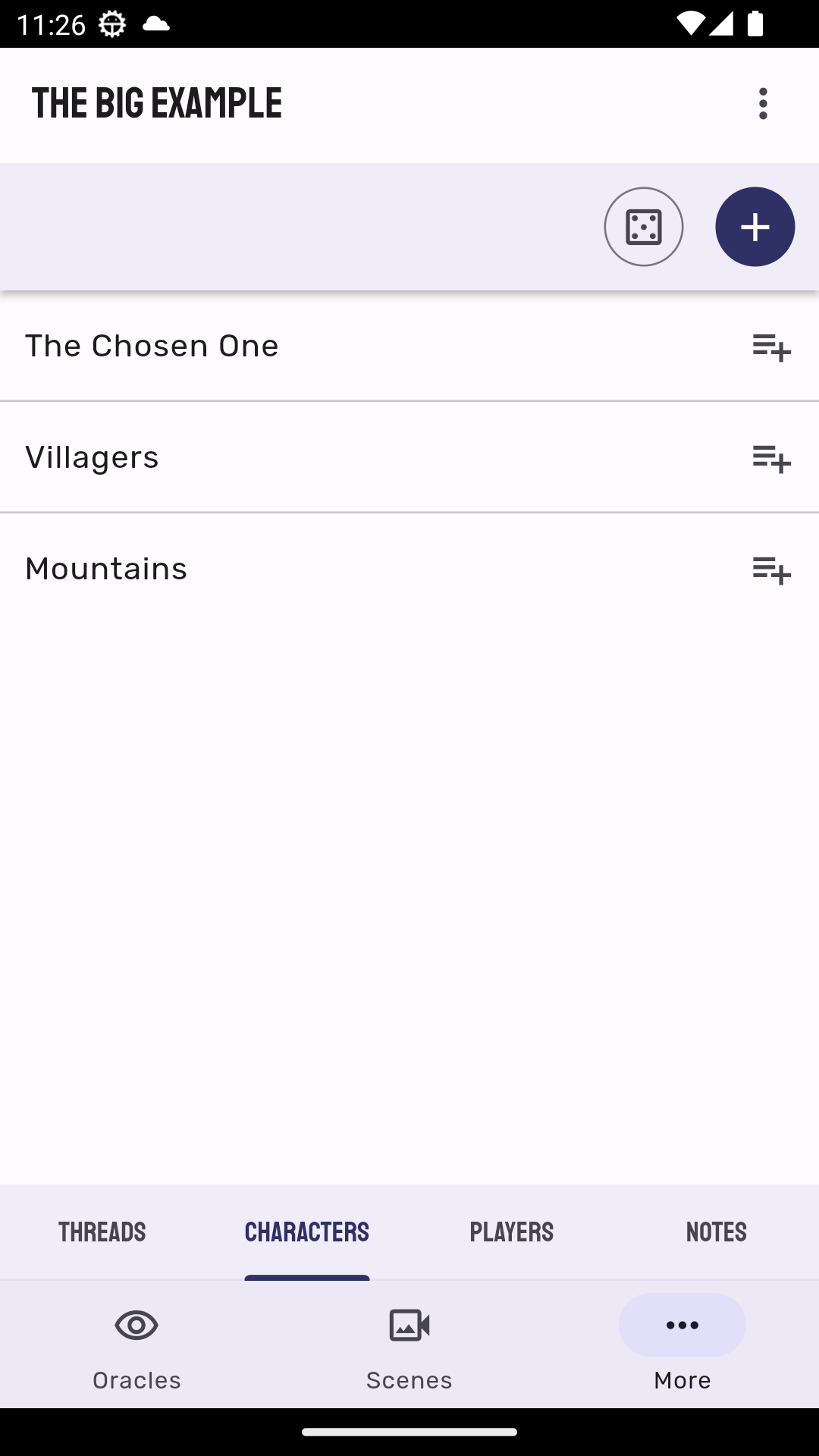Screenshot of a smartphone interface displaying a detailed fantasy role-playing game management screen. The status bar at the top shows the time at 11:26, a cloud icon, Wi-Fi signal strength, and battery level indicator. The main interface features black text on a light lavender background reading "The Big Example" with a menu button represented by three vertical dots on the far right. Beneath this, there are two circular icons: the left one displays a dice showing the number five, while the right one is a darker shade—either dark blue or dark purple—with a plus sign inside it.

Directly below these circles are three light lavender boxes labeled sequentially: "The Chosen One," "Villagers," and "Mountains." Each box has a set of three lines and a plus sign to their right, likely denoting options for adding or editing entries.

At the bottom section, there are two larger boxed tabs. The first one contains four tabs labeled: "Threads," "Characters," "Players," and "Notes," with the visible page being the "Characters" tab. Below this, there is an icon resembling an open eye labeled "Oracles," followed by additional labels "Scenes" and "More..." with an accompanying menu button represented by three vertical dots.

The interface is organized to manage and track various elements of a role-playing game, integrating character profiles, narrative elements, and other dynamic components essential for gameplay.